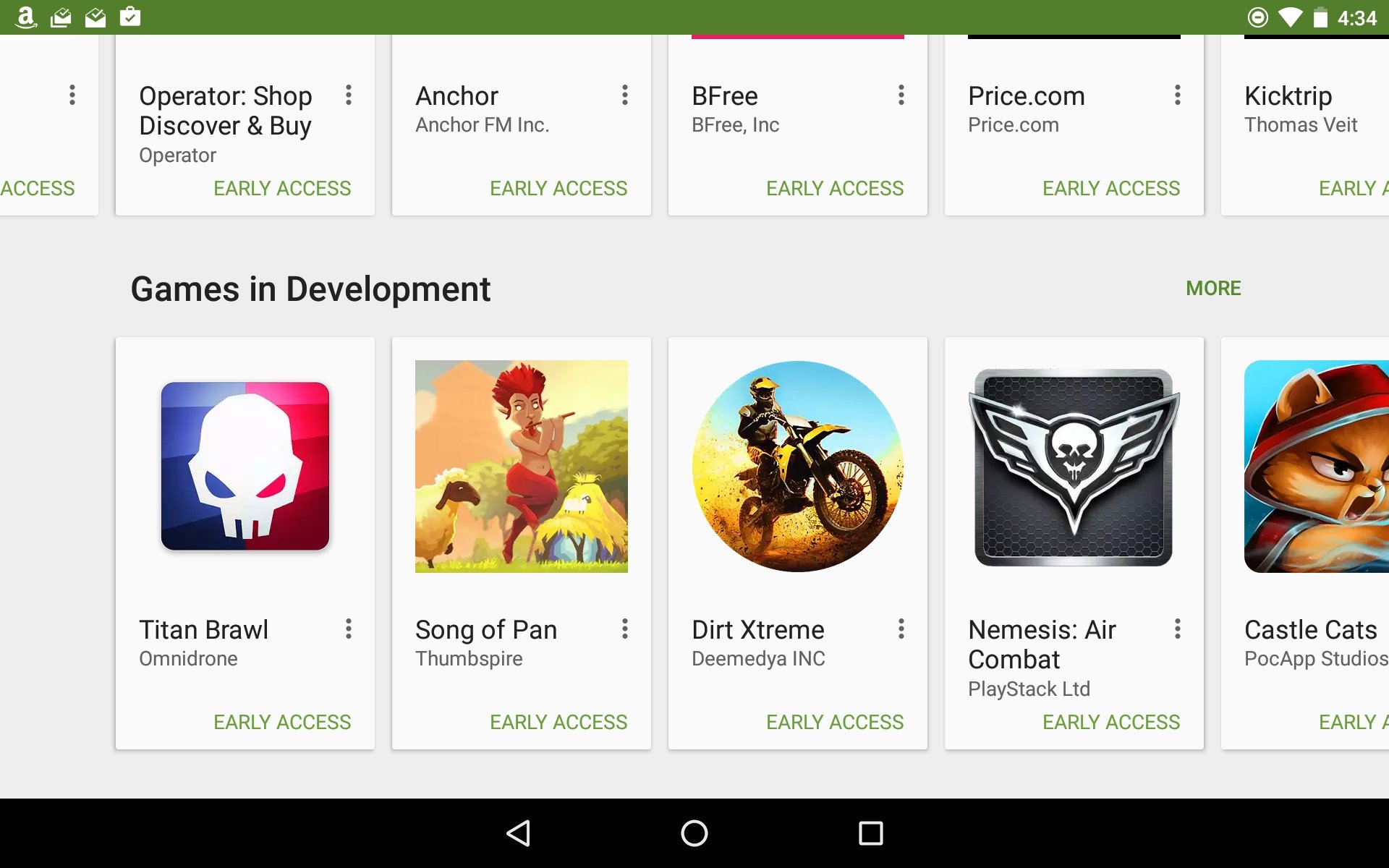This screenshot, presumably from a mobile device, displays an unfamiliar site overlaid by the browser header bar labeled 'WebsiteRab'. A prominent green banner spans the top of the page, featuring the Amazon logo and what appear to be various mail icons. The far right corner of the banner shows standard mobile interface symbols: time, Wi-Fi signal strength, battery level, and potentially location services.

Below the banner, six partially visible tiles are arranged in two rows. The furthest top left tile shows the word 'Access' alongside three dots for additional options. The adjacent tiles read 'Operator', 'Shop', 'Discovery', and 'Buy', each with 'Early Access' marked in green text and three dots for further interaction. The tiles on the right are labeled 'Anchor', 'Be Free', 'Price.com', and 'Kit Trip'.

Beneath these initial tiles is a section titled 'Games in Development', containing five more tiles. Each game is represented by its logo, additional options via three dots, and a green 'Early Access' tag. The games listed are: 'Titan Brawl', 'Song of Pan', 'Dirt Extreme', 'Nemesis Air Combat', and 'Castle of Cats'.